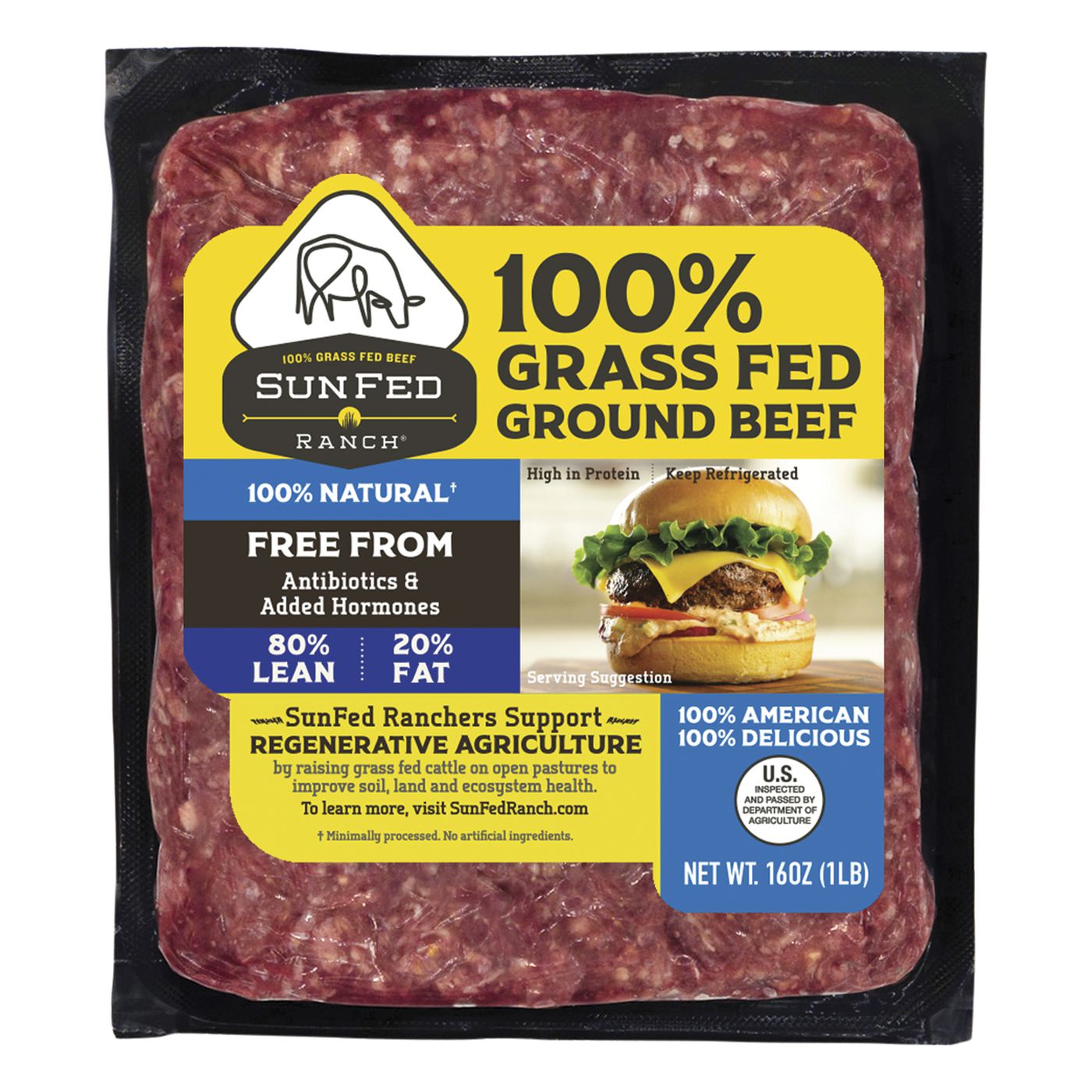The image depicts a vacuum-sealed package of ground beef, prominently showcasing its contents through a see-through plastic. The ground beef is encased within a black backing, which lends a stark contrast to the vibrant red of the meat, speckled with bits of white fat. Centrally located is a detailed sticker. At the top of the sticker is a black-and-white image of a cow, beside which the text “100% Grass-Fed Ground Beef” is emblazoned. Beneath this, a vivid depiction of a hamburger is visible, complete with bread, lettuce, cheese, a beef patty, tomatoes, onions, and a type of sauce.

The sticker also highlights key information: “100% Natural, Free from Antibiotics and Added Hormones, 80% Lean, 20% Fat, High in Protein, Keep Refrigerated.” The package bears the branding of SunFed Ranch, known for supporting regenerative agriculture by raising grass-fed cattle on open pastures to enhance soil, land, and ecological health. Further down, the sticker states, "SunFed Ranch supports regenerative agriculture," and provides a taste appeal with “100% American, 100% Delicious.” Addition details include “Net Weight: 16 oz (1 lb), U.S. Inspected and Passed by the Department of Agriculture,” and the URL “sunfedranch.com” for more information.

The colors on the sticker range from reds, whites, blues, blacks, and grays to yellows and greens, creating a visually engaging and informative label on the package.